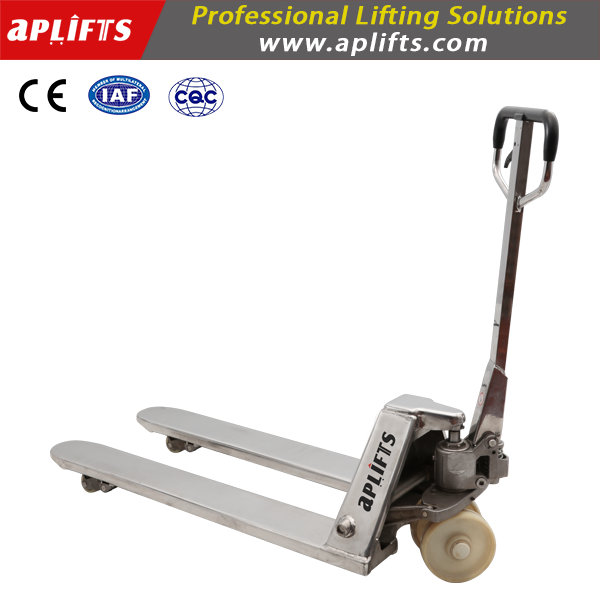The photograph showcases a forklift, prominently situated on a clean white background, appearing to be part of a marketing advertisement or website. At the top of the image, a banner in white text against a red background boldly displays "APLifts." Directly below, on a grey background, the text reads "Professional Lifting Solutions" in yellow letters, followed by the website URL "www.aplifts.com" in white letters. Beneath the banner are three certification logos: "CE" in black letters on a white background, "IAF" in white letters inside a blue oval outlined with a darker blue border, and "CQC" in white letters within a globe-like design. 

The forklift itself is metallic white or grey, designed for lifting pallets and similar objects. Key features include a silver-gray, adjustable handle situated in the upper right corner with a black trigger, white wheels located below the handlebar, and two protruding silver forks. The branding "APLifts" is visible on the side of the machine, incorporating a red dot over the 'i'. This detailed image highlights the functional and branded aspects of the forklift, emphasizing its professional application and certified standards.